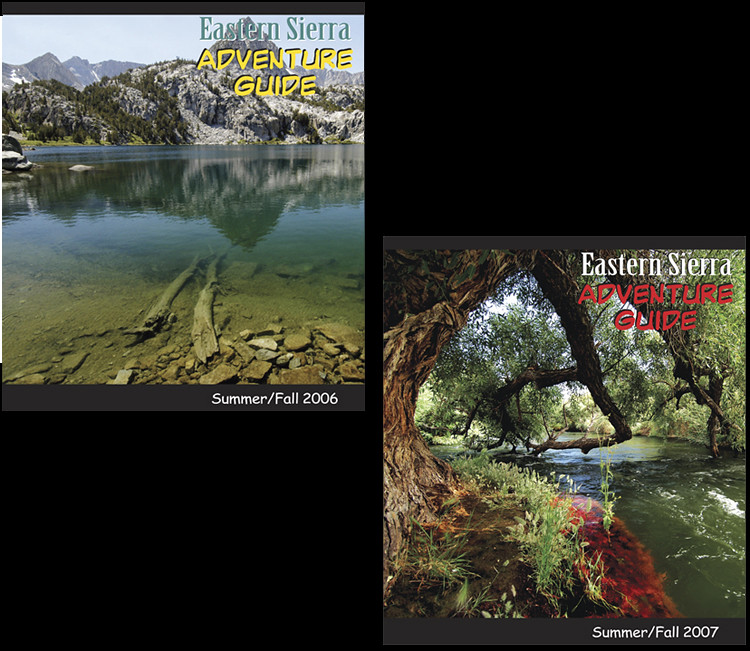This is a photograph showcasing two editions of the Eastern Sierra Adventure Guide from the summer and fall seasons of 2006 and 2007. The image features a large black background with two colorful photographs prominently displayed—one in the upper left corner and the other in the bottom right corner. 

The upper left photograph, from the Summer/Fall 2006 edition, captures a serene lake with a partly visible rocky sandy bottom. In the distance, a mountain range extends upwards, some peaks still dusted with snow, while others are bare of trees and grass due to their elevation.

The bottom right photograph, from the Summer/Fall 2007 edition, depicts either a small river or a large creek with visible white-capped water. The watercourse is flanked by large branches of trees that hang over, casting shadows on the water. Though the water is relatively calm, its depth is indeterminable, adding a sense of mystery and potential danger. The creek's bank is narrow and lined with grass and autumnal red foliage. Both images have the title "Eastern Sierra Adventure Guide" in the top right corner, with their respective edition years noted in the bottom right.